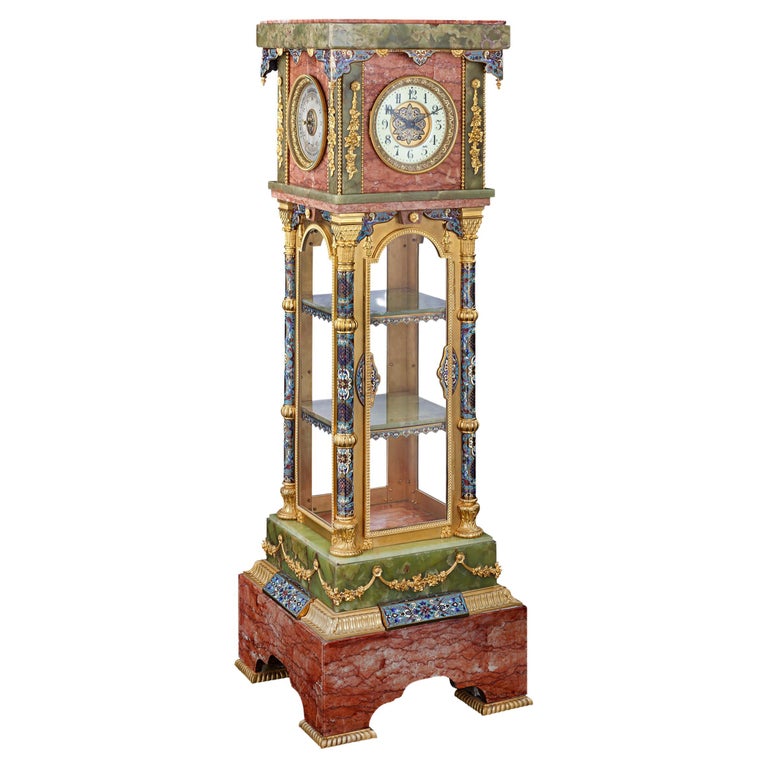This image depicts an intricately designed, ancient-inspired standing clock, reminiscent of a grandfather clock with potential Asian influences. The clock, made from a variety of materials including wood, marble, and jade, stands on a red marble base with dark veining and four gold-highlighted legs. The base transitions into a green jade block adorned with a gold element resembling a tiara. Above this, a rectangular section features glass doors and shelves, possibly for displaying items. Supporting the uppermost part of the clock are blue marble columns. The clock itself is situated within a red marble cube at the top of the structure. The clock face is predominantly white with blue numbers and hands, surrounded by intricate, ornate carvings and filigree in various colors such as green, red, blue, yellow, and gold. There are clock faces on at least two visible sides, each displaying standard numbers from 1 to 12, set against a red background. The overall design is highly detailed, with extensive use of ornate shapes and carvings on multiple parts of the structure.